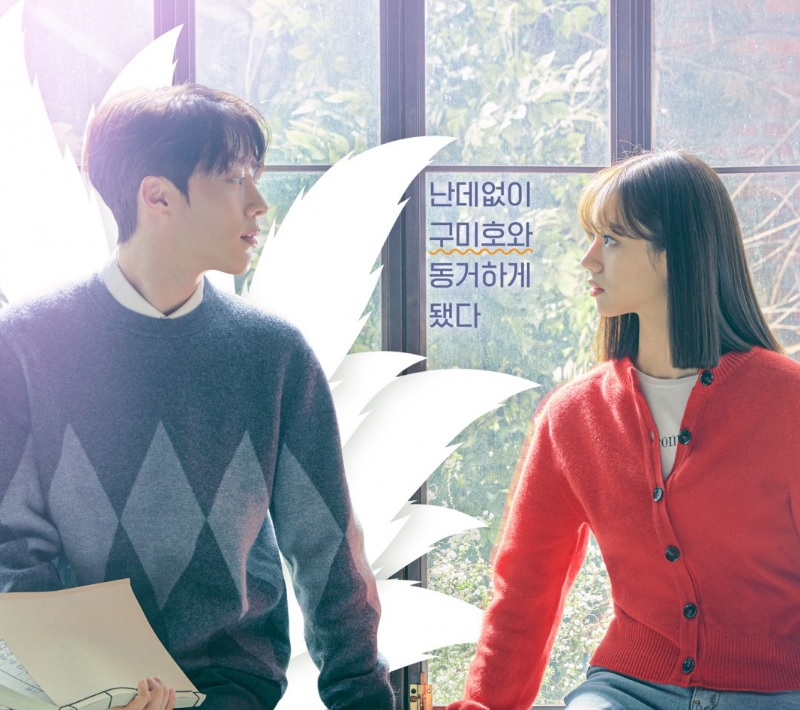The image depicts a scene reminiscent of a Korean or possibly Japanese rom-com, featuring a young Asian couple seated close together inside a bright room. The background is illuminated by sunlight streaming through a large window, which reveals green trees outside and casts a soft glow throughout the space. 

The young man, on the left, has dark hair and is dressed in a blue Argyle sweater, which features diamond shapes. He holds a manuscript or folder in his left hand, and has a white tail-like object behind him. The woman, on the right, is intently gazing into his eyes. She has straight, brown hair and brown eyes. She is wearing a red button-down sweater over a white T-shirt, paired with blue denim jeans.

Their faces are about two feet apart, but their shoulders are closer, approximately one foot apart, and it appears they may be holding hands just out of view. Behind them, the glass wall features some writing in an Asian script, possibly Japanese or Chinese, adding to the cultural ambiance of the scene.